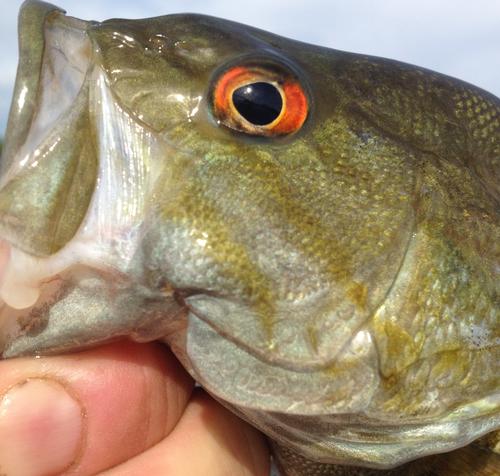This close-up photograph captures a recently caught fish being held by a person. The fish, with its greenish-gray body that transitions from dark green on top to lighter green and ultimately gray near its underside, stands out in vivid detail. Its scales exhibit variations in color, adding to the depth of the image. The fish's mouth is open wide, propped up by the person's fingers, possibly indicating that it was just caught. The fish's eye, striking with its red-orange hue and large black pupil, is wide open, reflecting the stark reality of a "fish out of water." The individual holding the fish has dirty fingernails, hinting at a recent fishing endeavor. The overall composition reveals the fish facing left, showcasing its gills and side body in sharp focus, while the absence of water further emphasizes its captured state.